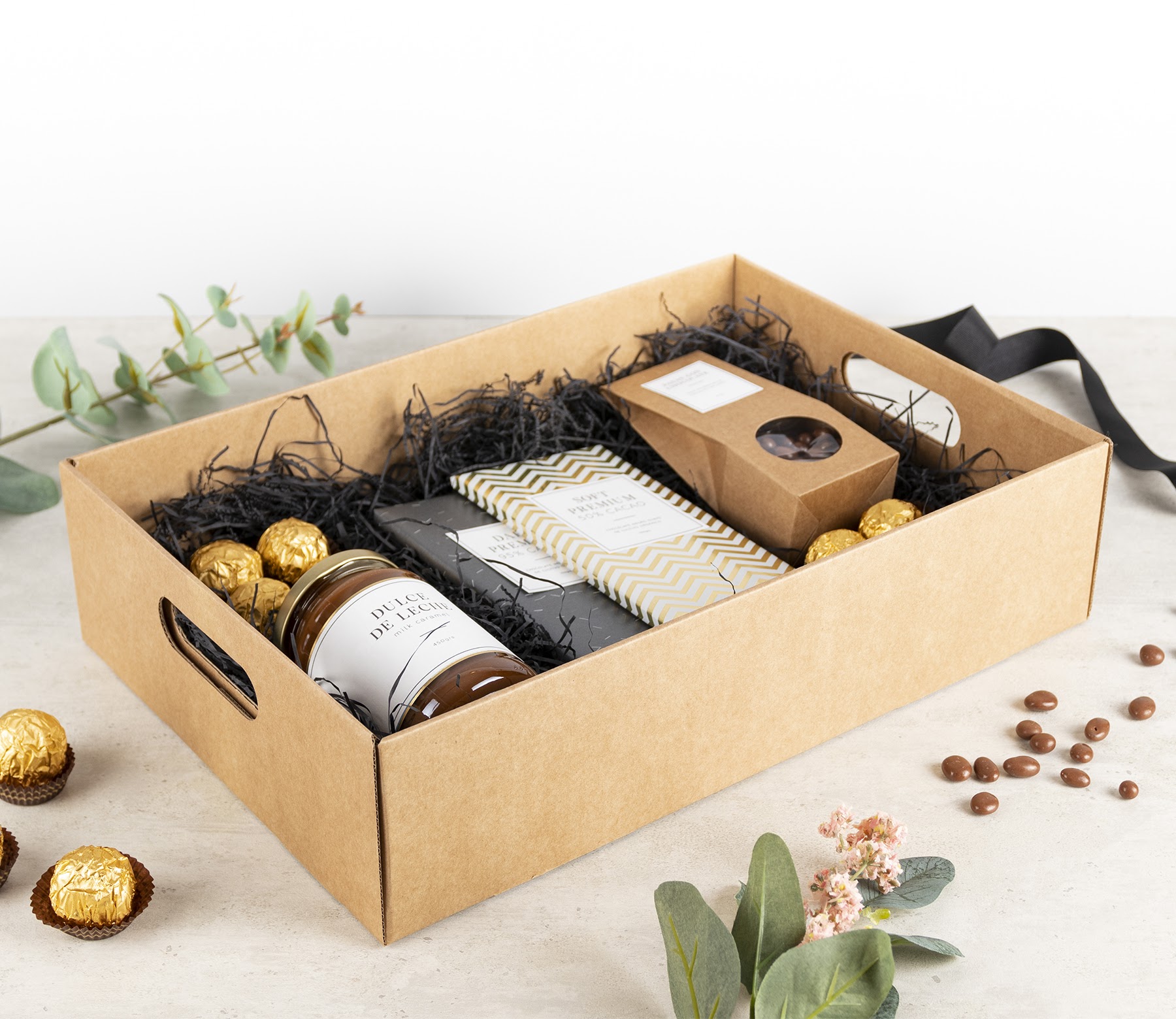The image showcases an aesthetically arranged gift box on a light tan table, set against a white wall. The gift box, made of cardboard and adorned with a ribbon, is nestled among decorative black confetti and is surrounded by a strand of faux eucalyptus leaves and small pink flowers both at the top and bottom corners. Scattered on the table are Ferrero Rocher chocolates, identifiable by their gold foil wrapping, and small chocolate-covered raisins or brown pebble-shaped candies. Inside the box, prominently placed on the left, is a jar of Dulce de Leche with a white label, rich caramel liquid visible through the glass. In the center are two neatly placed chocolate bars, and on the right, a brown decorative bag with a clear window filled with more chocolate-covered raisins. The overall setup, likely part of a marketing campaign, exudes a luxurious and gourmet presentation, ideal for attracting attention on social media platforms like Instagram.